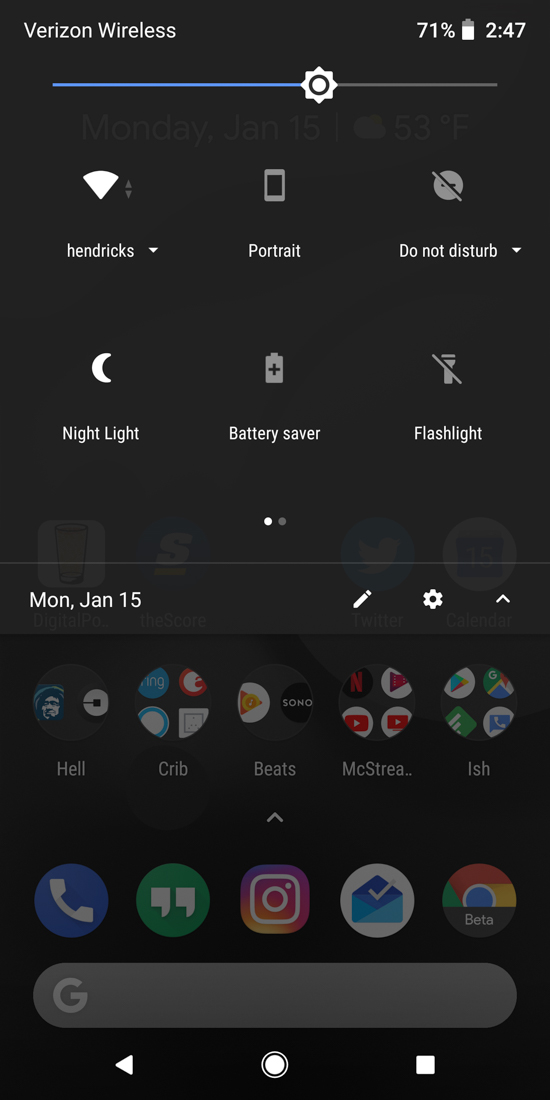The image showcases a screenshot of a mobile device, likely a cell phone or tablet, operating on the Verizon Wireless network. The status indicators at the top reveal a battery life of 71% and the time set at 2:47 PM. The device is utilizing a dark theme, as evidenced by the predominantly black background and white text.

At the top of the screen, the settings menu is open, displaying a brightness adjustment bar and various toggles for features such as Wi-Fi, Portrait Mode, Do Not Disturb, Night Light, Battery Saver, and Flashlight. The date is noted as Monday, January 15th. Icons for editing, accessing further settings, and closing the menu are also visible.

In the background, beneath the settings overlay, part of the device's home screen can be seen. It includes commonly used app icons, such as Google Chrome, a mail application, and Instagram. A gray Google search bar is situated near the bottom of the home screen, and navigation buttons for Back, Home, and Recent apps are aligned at the very bottom.

Additionally, several app groupings are labeled with titles such as "Hell," "Crib," "Beats," and "Ish," suggesting categorical organization for the user's apps.